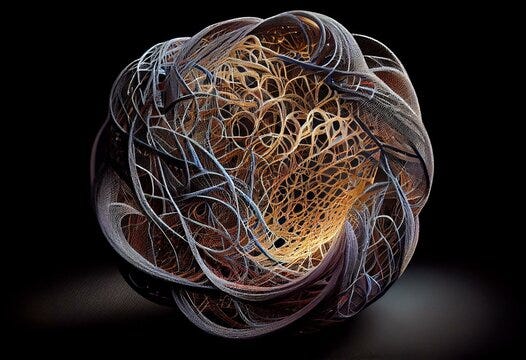The image portrays an artistic, computer-generated rendering or possibly an abstract sculpture, set against a solid black background. It features a complex arrangement of continuous, spaghetti-like lines forming a convoluted, somewhat spherical structure. The outer strands exhibit dark gray to creamy pink-gray hues, while the internal lines glow with a lighter shade, ranging from whitish-cream to light gold or beige. The object is evenly illuminated from above and within, casting subtle shadows on the black surface beneath it. Its wavy, intertwined lines create a mesmerizing pattern of whirls and swirls, suggesting an abstract, decorative piece that dominates the entire frame with no other elements present.